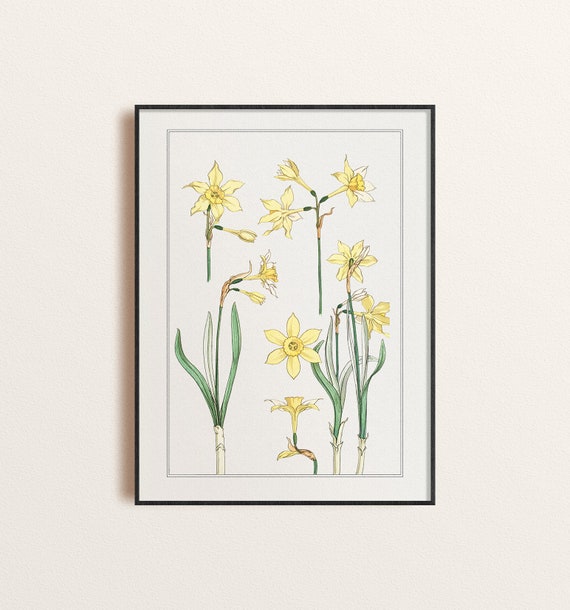The image displays a floral illustration mounted on a pristine white wall. The artwork is enclosed within a slender black rectangular frame, oriented vertically. The illustration features multiple renditions of daffodil-like flowers, primarily characterized by their six yellow petals and round centers. 

Starting from the top, two green stalks, one showcasing a fully bloomed daffodil and the other displaying a budding flower, are depicted. Moving to the left side, there are two additional flowers with long green leaves, while the right side portrays three flowers growing from a single stem. The bottom section illustrates several stalks emerging from the ground, exhibiting a mix of blooms and buds, accompanied by elongated green leaves. The detailed portrayal captures the various growth stages of the daffodils, emphasizing their vibrant yellow petals contrasted against the greenery.